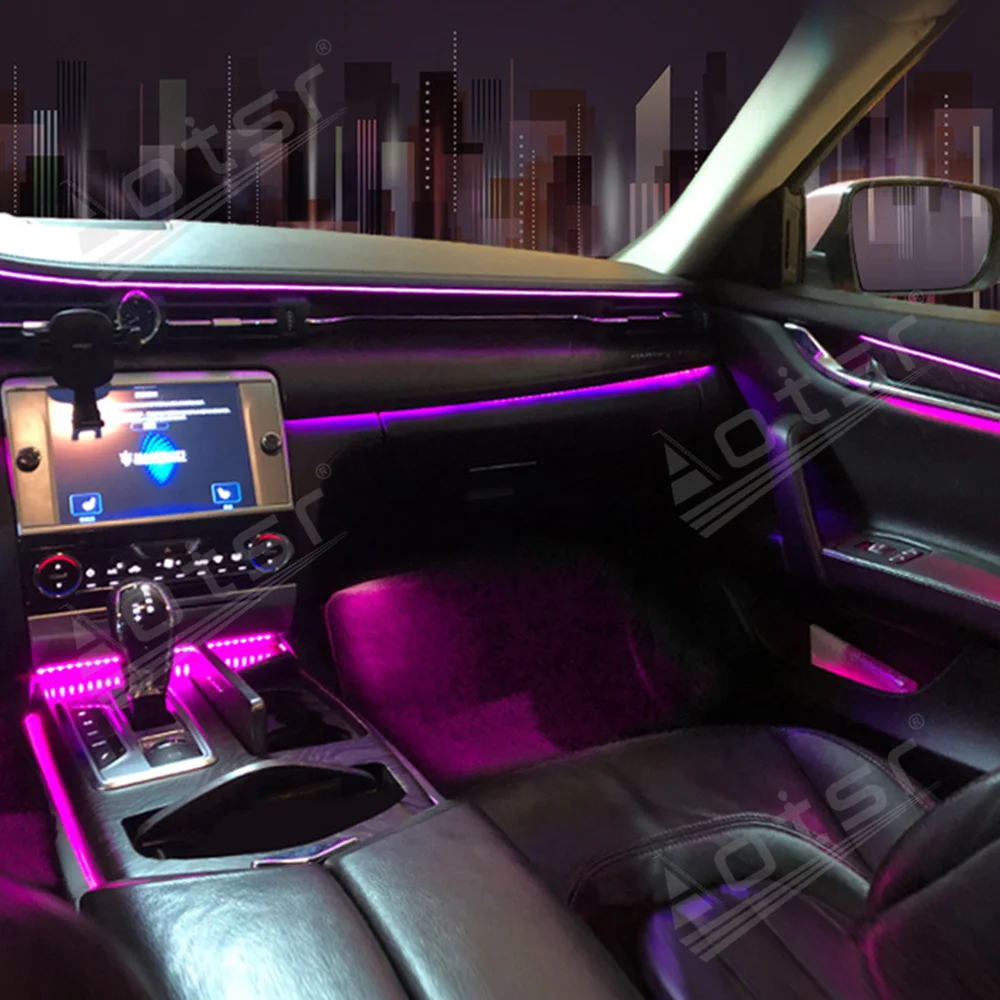The image is a color photograph capturing the interior of a car with a highly detailed and futuristic design. The car interior features black leather seats and a matching black leather console. Prominent in the semi-blurry shot is a black and silver gear shift, a large blue digital LED screen on the front console with blurry white text, and two silver knobs flanking the screen. Below it, the air conditioning controls comprise two knobs—red on top, blue on the bottom—and multiple buttons in the center. The dashboard is a hard light gray material, illuminated by striking purple ambient lights that cast a glow over the console and floor. The passenger door, visible with a white piece of paper in the cubby, also gleams with the same purple light. Through the car’s windshield and passenger window, a synthetic, digital cityscape can be seen under the cover of night, adding to the surreal and futuristic ambiance of the photograph.